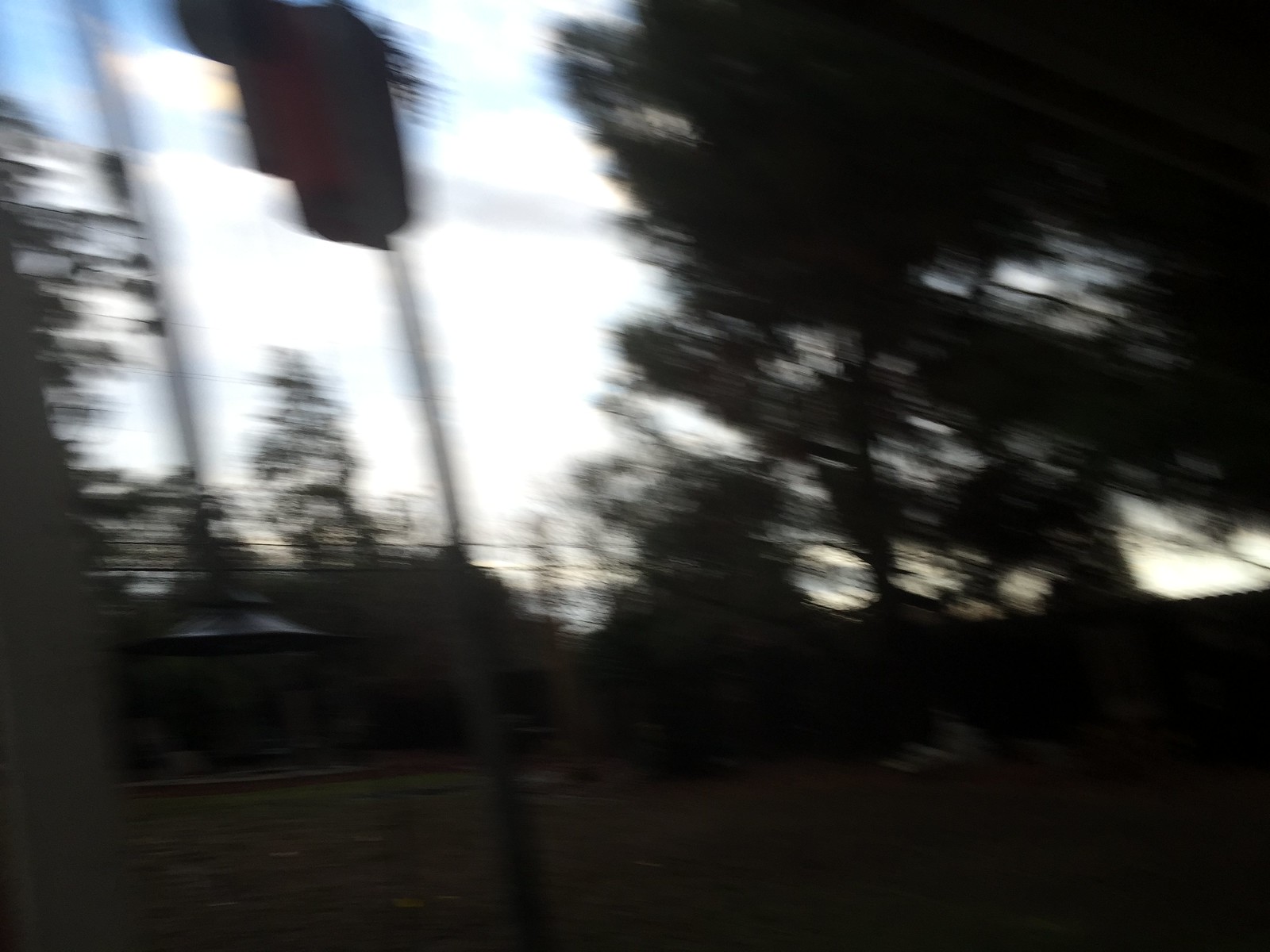A photograph taken during the serene moments of sunset or sunrise captures the tranquil ambiance of a park shrouded in a veil of motion blur. At the heart of the scene, a slightly discernible gazebo stands amidst a plentiful array of shadowy trees, their leaves merging into the encroaching darkness. The ground shares the same obscurity, blending seamlessly into the dim environment, thus, erasing any distinct features. Scattered sporadically, faint outlines of objects—potentially light poles or telephone poles—contribute to the park's mysterious atmosphere. Overhead, the sky provides a gentle contrast with patches of white and blue peeking through the darkened canopy. Pathways, barely visible, weave around the gazebo, guiding the eye through the hushed, enigmatic park.